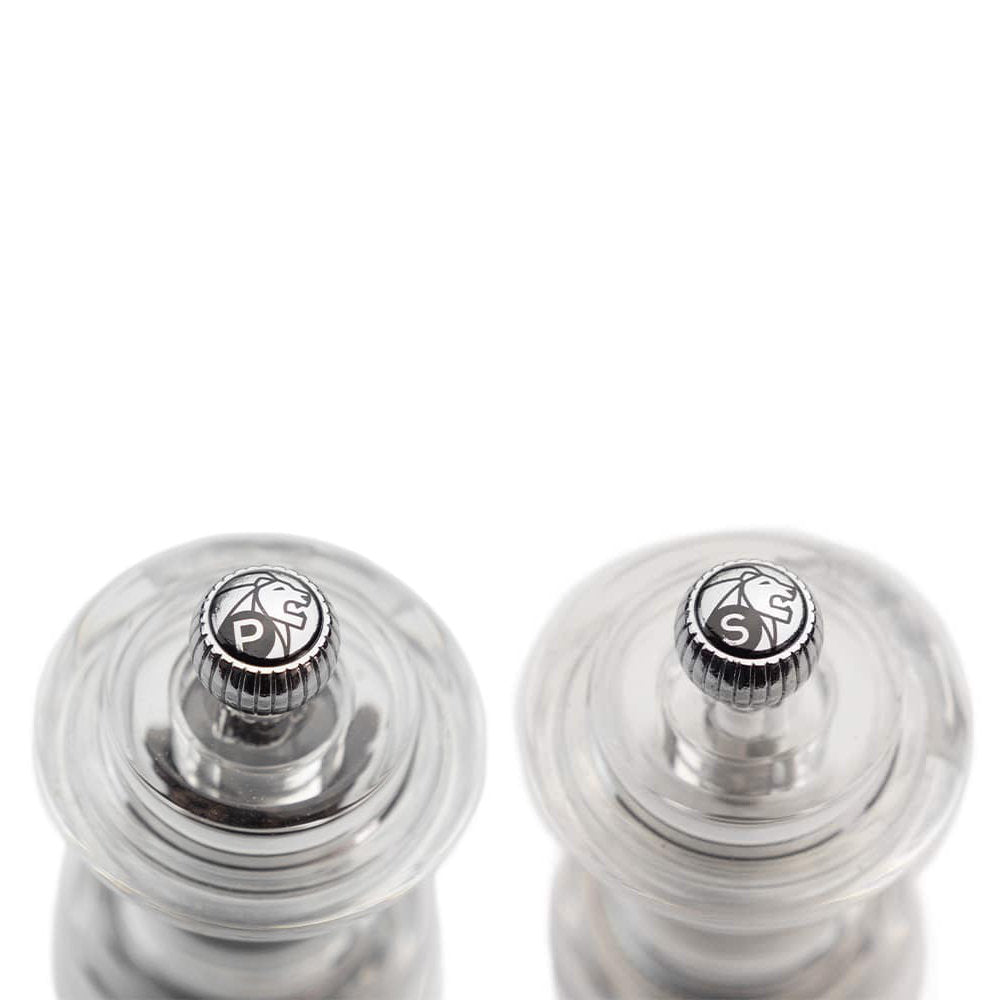This close-up photograph captures a pair of sleek, transparent salt and pepper shakers standing against a completely white background. Each shaker is topped with a shiny silver knob that features ridged sides and a simple black outline drawing of a lion. The shaker on the right has an "S" in a small black circle, denoting salt, while the one on the left has a "P" in a similar black circle, indicating pepper. Though the white background camouflages the contents of the salt shaker, the clear glass reveals whole black peppercorns inside the pepper shaker. The distinct, detailed design elements, like the lion drawings and the marked caps, showcase both functionality and aesthetic appeal, making these shakers suitable for both a home kitchen or a restaurant setting.